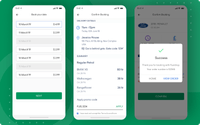The image features three smartphones displayed against a solid green background. Each phone is shown with a mostly white screen, though the text on them is largely indiscernible. The phone on the far right stands out due to a prominent white square in its center, within which the word "SUCCESS" is clearly visible. It is grayed out except for this word, and there is a green checkmark at the top of the white square. Additionally, this phone screen shows green square bars at the bottom, beneath the white square. The text across all three screens appears to be in black, but the specific details are difficult to make out. Overall, the image seems to emphasize the successful status indicated on the right-most phone.